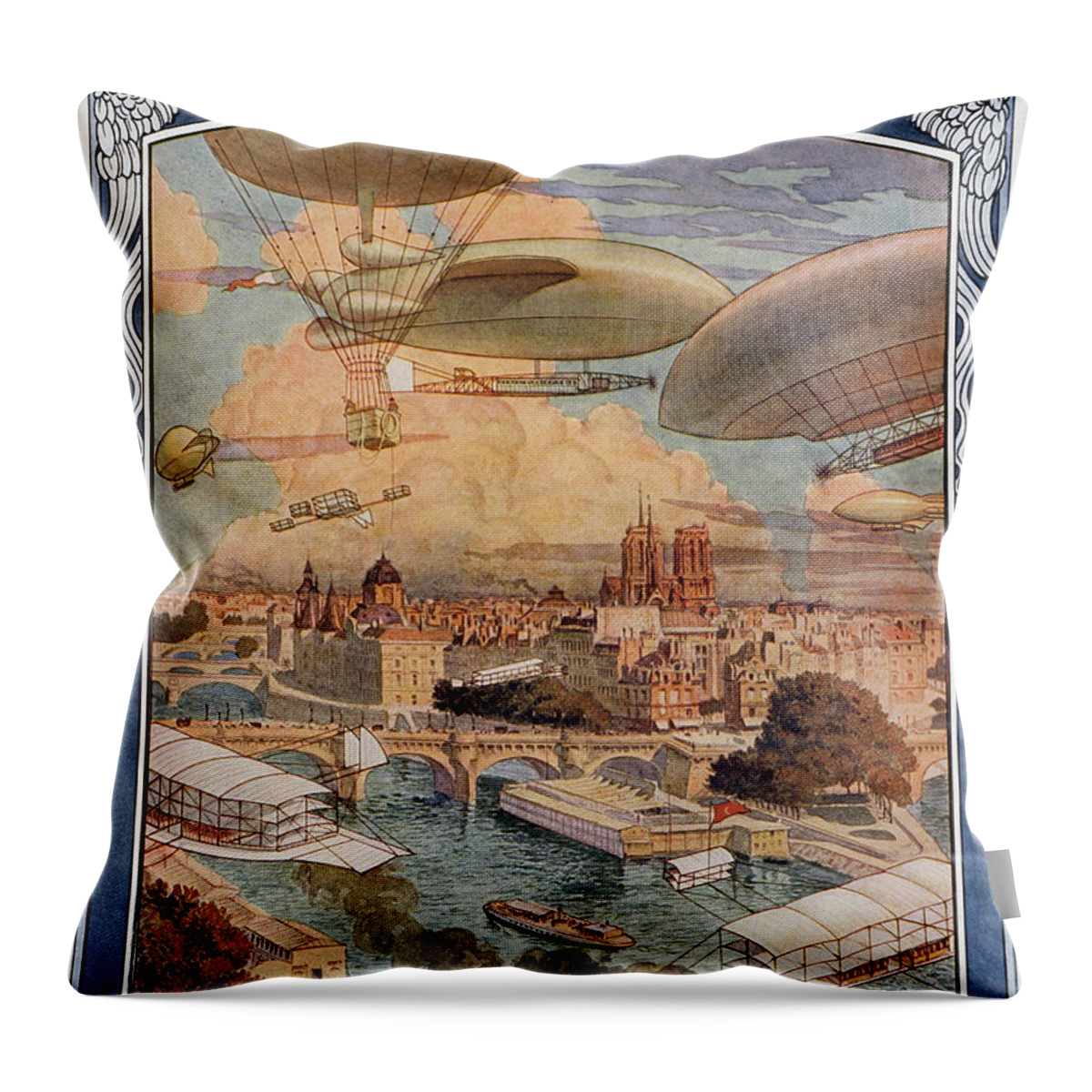This product image features a detailed vintage-style throw pillow set against a plain white background, ideal for showcasing its intricate design. The pillow's artwork, reminiscent of a Jules Verne novel, portrays a bustling sky filled with bullet-shaped airships and hot air balloons, each with wire-framed carriages reminiscent of early aviation. Among these is even a historic Wright Brothers airplane. The aerial scene unfolds over an Italian or European-inspired city, evocative of Venice, with its numerous canals, bridges, and distinctive plaster-cement buildings. Boats of various types, including sailboats, float on the waterways, adding to the lively old-world charm. The background of the image features a blue sky, enhancing the vintage allure of the scene, possibly designed with pulp magazine aesthetics in mind.